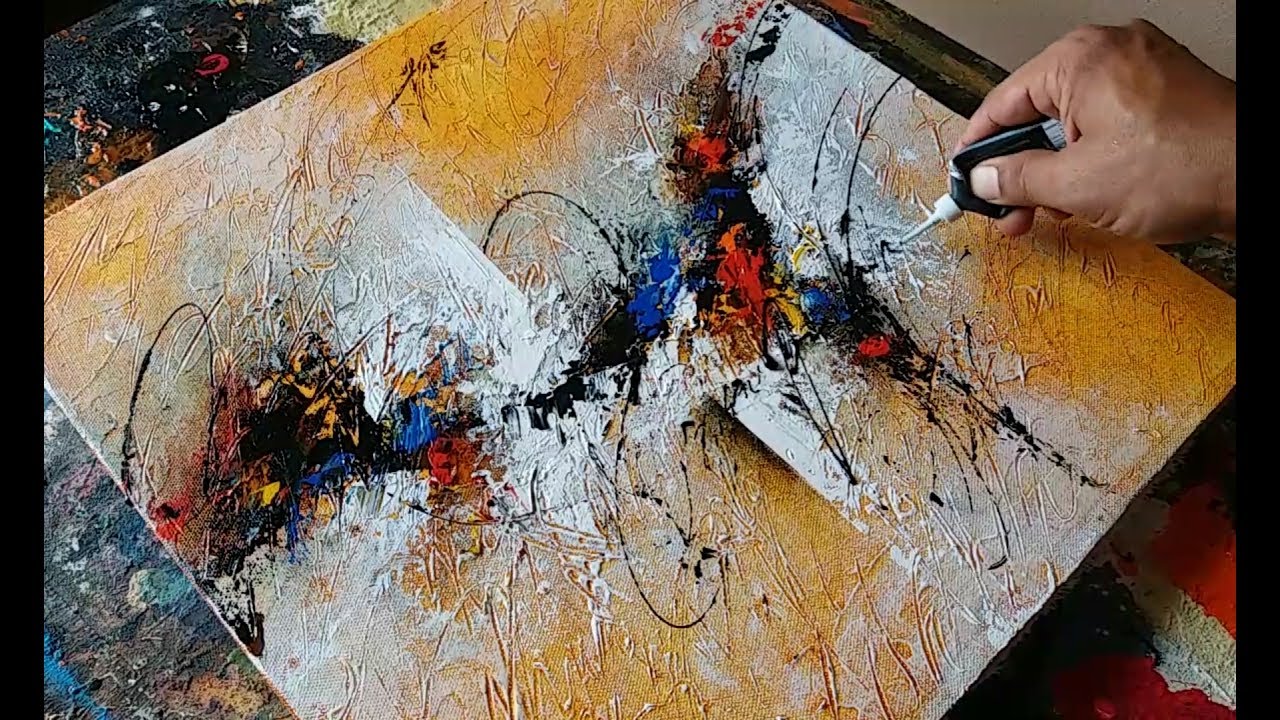An overhead view captures an artist engrossed in their work on a sprawling canvas that dominates the image, its corners extending beyond the frame. The canvas rests on a well-used, paint-splattered table, revealing the creative chaos of the workspace. The artist's right hand is visible, firmly squeezing a tube of paint through a white nozzle, adding to their abstract creation. The canvas itself features a tan background, intricately adorned with random patches of white. Cutting through the center is a vibrant, chaotic band of colors—blues, reds, oranges, and yellows intermingled with stark black streaks, lending a sense of dynamic movement to the composition. The overall design is abstract and non-representational, reflecting an unbound, expressive artistic process.